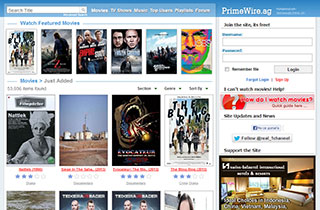The screenshot is of a website titled "Primewire.ag," prominently displayed in the upper right corner. The top corner of the screen features a lighter blue row that spans across. In the far left corner of the blue toolbar, there is a search bar, followed by the text "Movies" and "TV shows." Some of the text to the right is too faint to discern clearly, but the website appears designed for watching movies and TV shows.

Just below the search bar in the upper left, there is a row of five movie posters under the headline "Watch Featured Movies." Further down, there is another section labeled "Just Added," showcasing newly added movies. The right third of the screen is dedicated to a column that starts with a login section at the top, followed by a series of advertisements occupying the lower portion. The layout and various sections of the website suggest a user-friendly interface focused on providing access to a wide range of movies and TV shows.